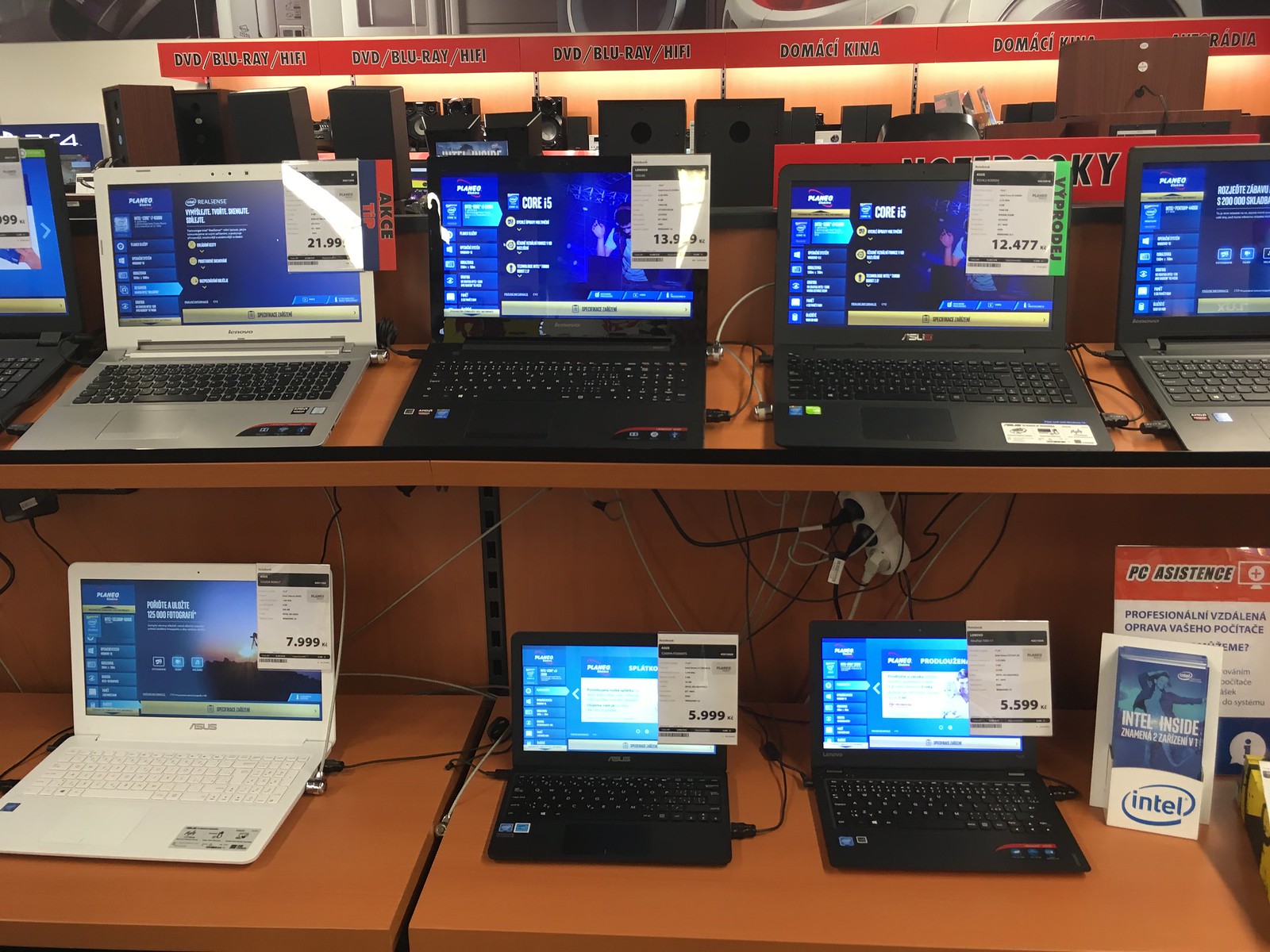The photograph captures a display in a retail electronics store, specifically focused on showcasing several laptops. Positioned on two orange wood shelves, there are a total of seven open laptops. Each shelf holds multiple laptops, with the lower shelf housing three fully visible and the upper shelf holding four, though only partially within the frame. All the laptops are operational with their screens illuminated, displaying what appears to be a start page with identifiable but unreadable fine text on the left sidebar and a prominent square in the middle of the screen. Attached to the displays are price tags, with the prices ranging from approximately $5,000 to over $12,000. Additionally, a brochure reading "Intel" is propped up beside one of the laptops. In the background, the store includes additional electronics such as speakers and has posters and a lighted display on the walls. The textual detail and pricing suggest the store may be located in an Eastern European country, inferred from the styling of the text on the price tags.